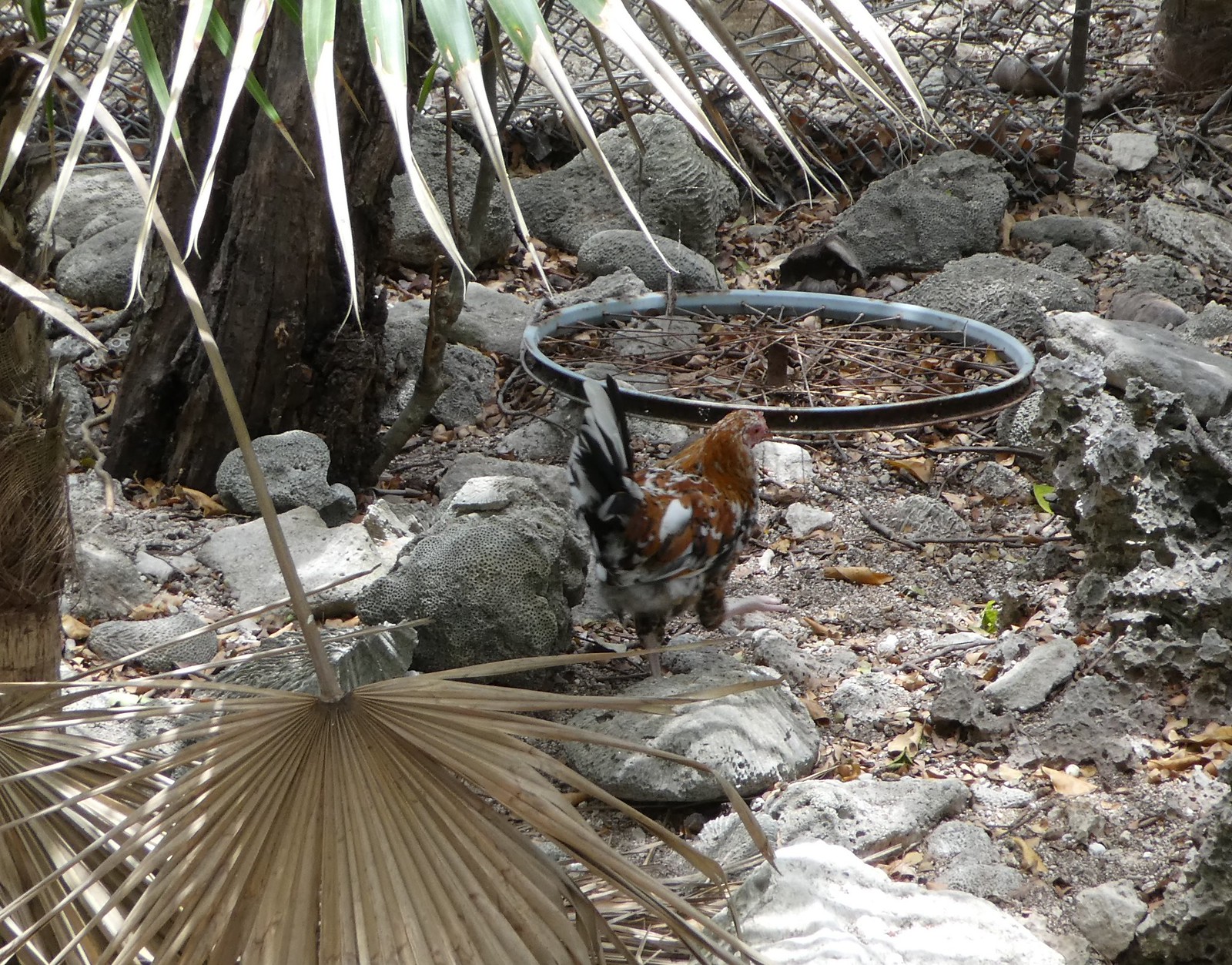In this outdoor image, a brown, black, and white chicken, possibly a rooster, stands amid a cluttered, rocky environment. The ground is scattered with numerous gray stones, pebbles, and brown leaves, giving the area a rugged appearance. Sunlight illuminates the scene, enhancing the colors of the surrounding greenery and the weathered elements. To the right of the chicken, an old bicycle wheel, white on the inside and black on the outside with rusted spokes, lays discarded among the rocks and debris. The background is dotted with tropical plants, including dried, fan-shaped leaves that resemble palm fronds, and the base of a brown, weathered tree that looks dark and possibly wet. Long, skinny, light-green leaves, like daggers, protrude from the top of the image, contributing to the tropical feel of the setting.